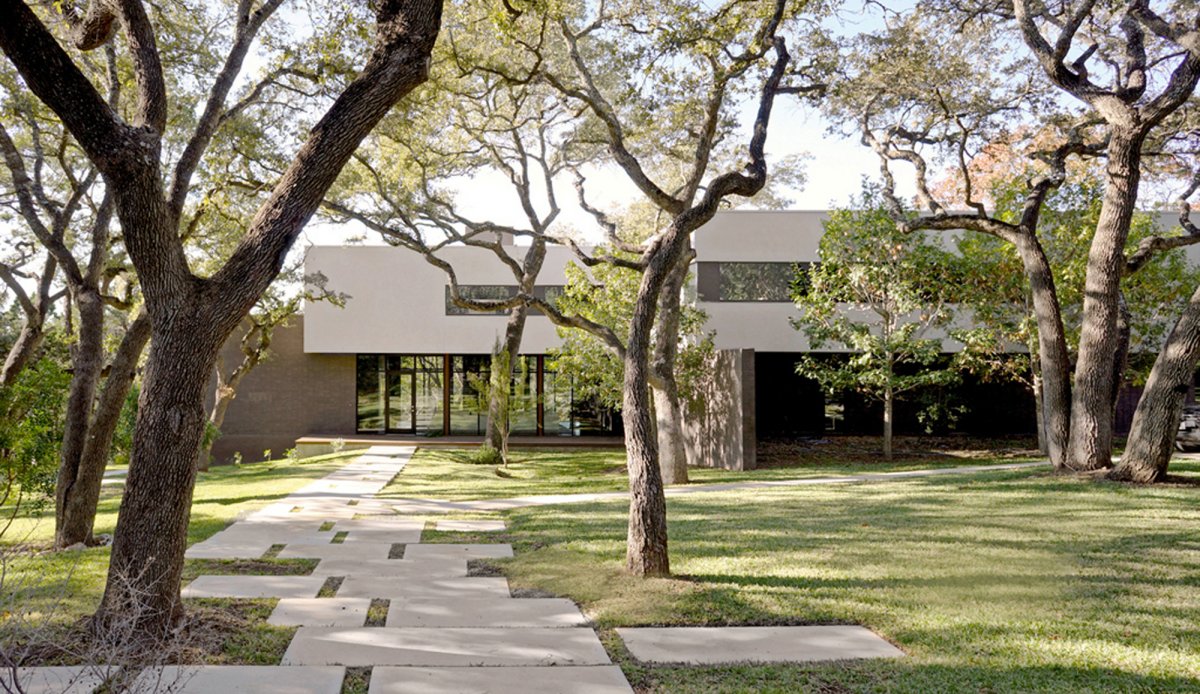This image captures a modern-looking, potentially multipurpose building, possibly a house, office, or school, set in a lush outdoor environment on a sunny day. The structure features a combination of tan and silver surfaces, with a distinctive silver roof adorned with skylights. One notable characteristic of the building is the expansive use of glass; an entire room at the front appears to be made of windows, showcasing an open, airy feel.

The façade of the building includes three sets of glass doors to the left, indicating possible entry points. In front of the building, there is a meticulously designed concrete sidewalk consisting of square slabs laid out in a pattern. This pathway is not strictly linear but rather jagged, with cutouts that allow grass to peek through, leading directly to the front doors.

The surrounding landscape is dotted with mature, somewhat sparse trees, which frame the main entrance and extend along the sidewalk. Some of the trees display hints of fall colors, with a few leaves turning red or orange, contributing to the overall natural and serene aesthetic. The grass on the lawn is lush and green, although a few sticks are visible, particularly to the bottom left of the image.

Above the building, the sky is a light blue, peppered with fluffy white clouds, enhancing the bright, clear atmosphere of the scene. Overall, this detailed portrayal emphasizes both the architectural elements and the harmonious integration of nature in the setting.